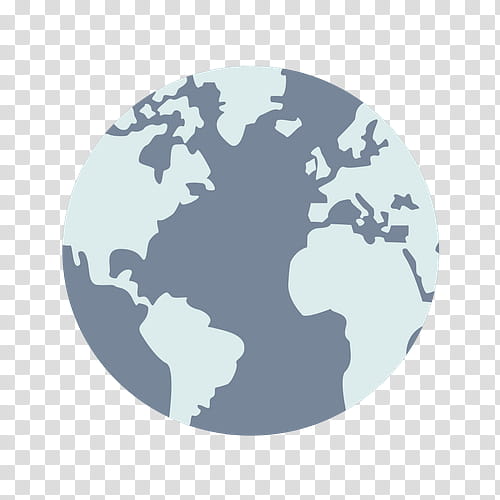This detailed vector artwork illustration depicts a cross-section of the Earth, showcasing parts of the United States, South America, Africa, a portion of Europe, and Greenland at the top. The landmasses are rendered in a light, grayish-blue hue, while the oceans are a darker gray, contributing to a somewhat faded and muted overall color palette. The globe itself is set against a transparent background with a pale checkerboard pattern that alternates between white and a very light blue, becoming more faded towards the bottom. The drawing style is notably rough, meaning the landmasses, though recognizable, are not intricately detailed but rather roughly sketched.